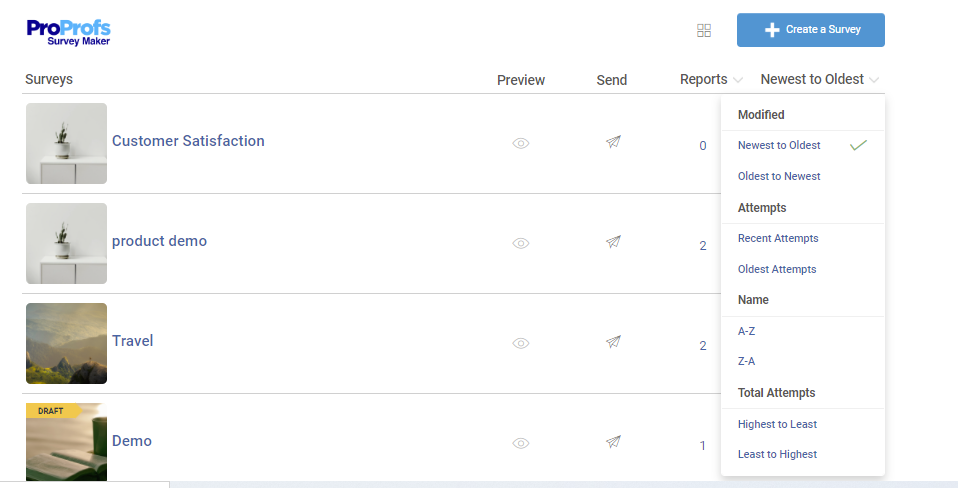On the web page, displayed in the upper left-hand corner, the text "Pro" is rendered in dark blue font, followed by "Profs" in light blue font. Directly beneath this text, the word "SurveyMaker" appears in the dark blue font used for "Pro." 

The main content area is organized into four categories listed vertically. These categories are labeled, from top to bottom, as "Customer Satisfaction," "Product Demo," "Travel," and "Demo," all in gray font. 

In the upper right-hand corner, there is a rounded rectangular button with a white plus sign and the text "Create a Survey" in white font. Directly below this button, a dropdown menu is indicated by a light gray downward caret, beside the text "Newest to Oldest" in black font and another light gray arrow. 

Further down, there is a vertical rectangular box displaying several options for sorting. From top to bottom, the options are "Modified" in black text, "Newest to Oldest" with a check mark on the right side in dark blue text, "Oldest to Newest" in dark blue text, and "Attempts" in black text, indicating a new category. 

A horizontal light gray line separates these options from the following: "Recent Attempts" and "Oldest Attempts" in the same dark blue font. Below these, there are additional alphabetical sorting options: "A through Z" in black text followed by a horizontal line under "Name," and "Z through A" in dark blue text. Lastly, the category "Total Attempts" is highlighted in dark black text, followed by sorting options "Highest to Least" and "Least to Highest" in dark blue font, separated by another horizontal line.